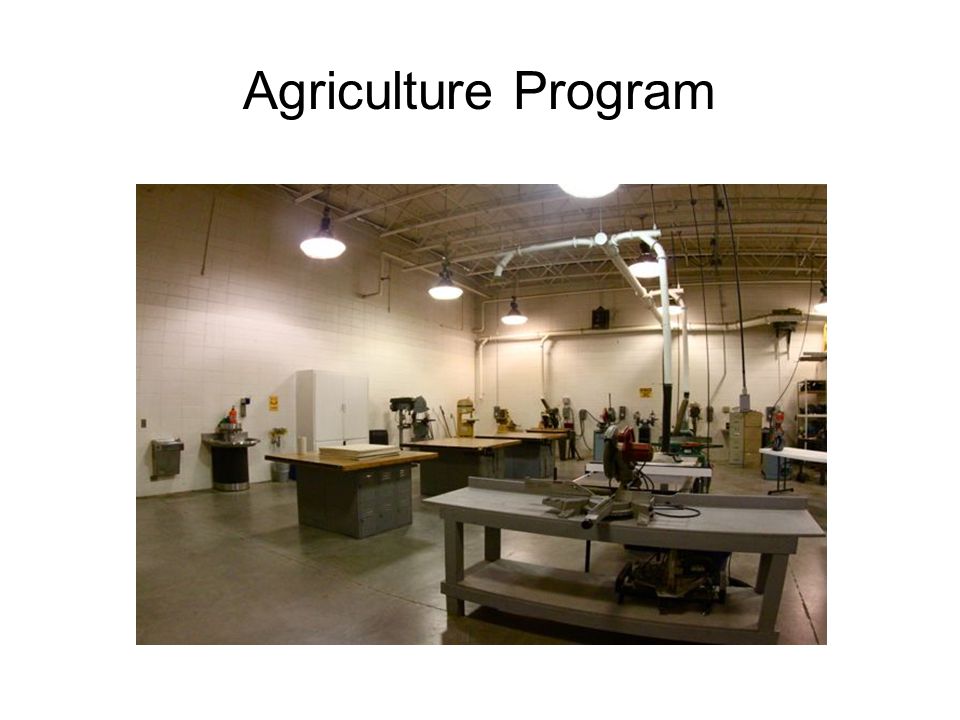The image captures the interior of an expansive, high-ceilinged workshop, labeled as part of an "Agriculture Program" in prominent black text at the top of the frame. This industrial space is well-equipped with multiple workbenches and tables, displaying an array of cutting and measuring tools. Notably, a long plastic table on the right is cluttered with equipment both on its surface and on a shelf beneath it. A distinctive wooden table with a concrete base stands out in the center, surrounded by various tools and projects in progress. 

The ceiling reveals exposed pipework and ductwork alongside a network of metal lattice structures. Hanging from the ceiling are large utility lights—seven in total—casting bright illumination across the room. A remote control lever dangles from above, typically used for maneuvering substantial machinery. On the left side of the image, a black trash can and a white cabinet accompany a wall-mounted water fountain, adding to the functional aspects of the workspace. Despite the bustling setup, the room is devoid of people, emphasizing its readiness for action without current activity.